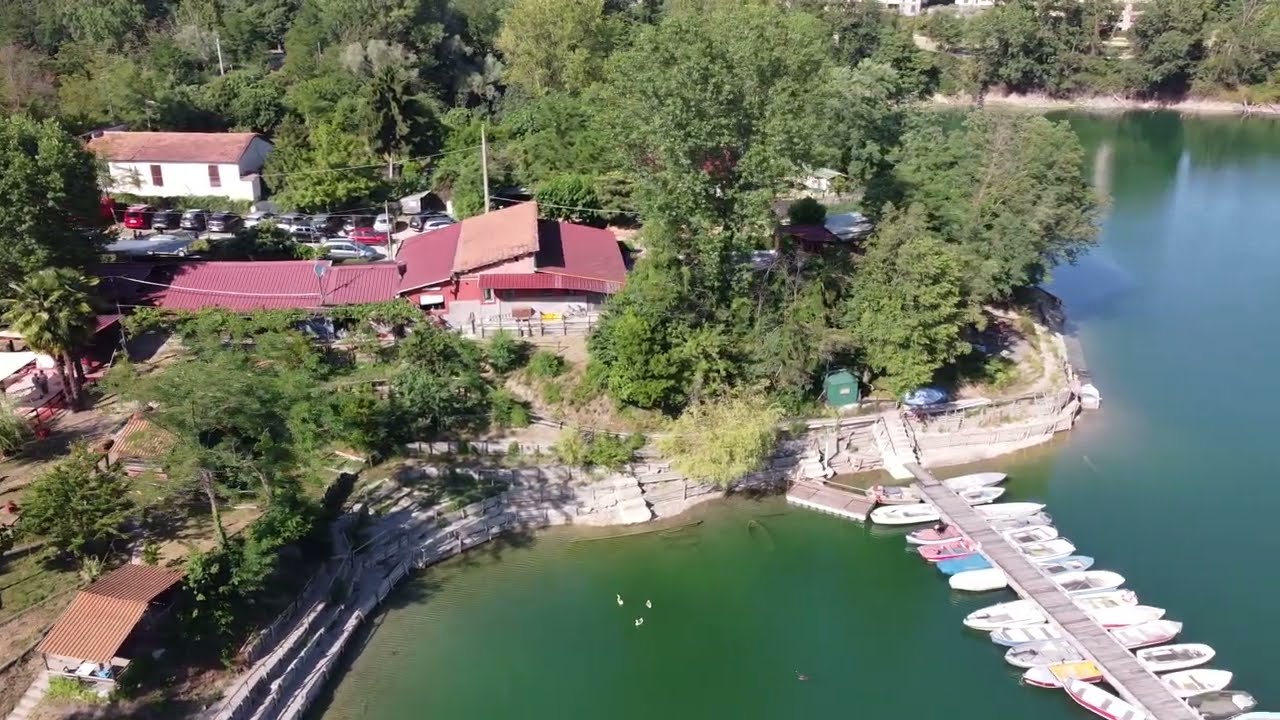The photograph, taken from high above, possibly by a drone, captures an idyllic small town nestled alongside a body of water, reminiscent of a quaint lakeside neighborhood. Dominating the scene is a long dock extending from the land into the water, where approximately 20-25 colorful rowboats—white, pink, red, blue, and yellow—are neatly tied up, creating a vibrant tableau against the serene lake. Adjacent to the dock, the shoreline forms a small cove, adding to the picturesque charm. The image also includes three seagulls leisurely floating near the dock, while a few objects, possibly people, can be discerned in the water below the dock. Stepping stones connect the waterfront to the land, where a cluster of buildings with striking red-tiled roofs can be seen amidst an abundance of large trees. A notable building just above the dock features a distinct red roof and is surrounded by other structures, creating a cozy, neighborhood ambiance. A large parking lot filled with cars is visible behind these buildings, indicating the area is a bustling docking port of the town.